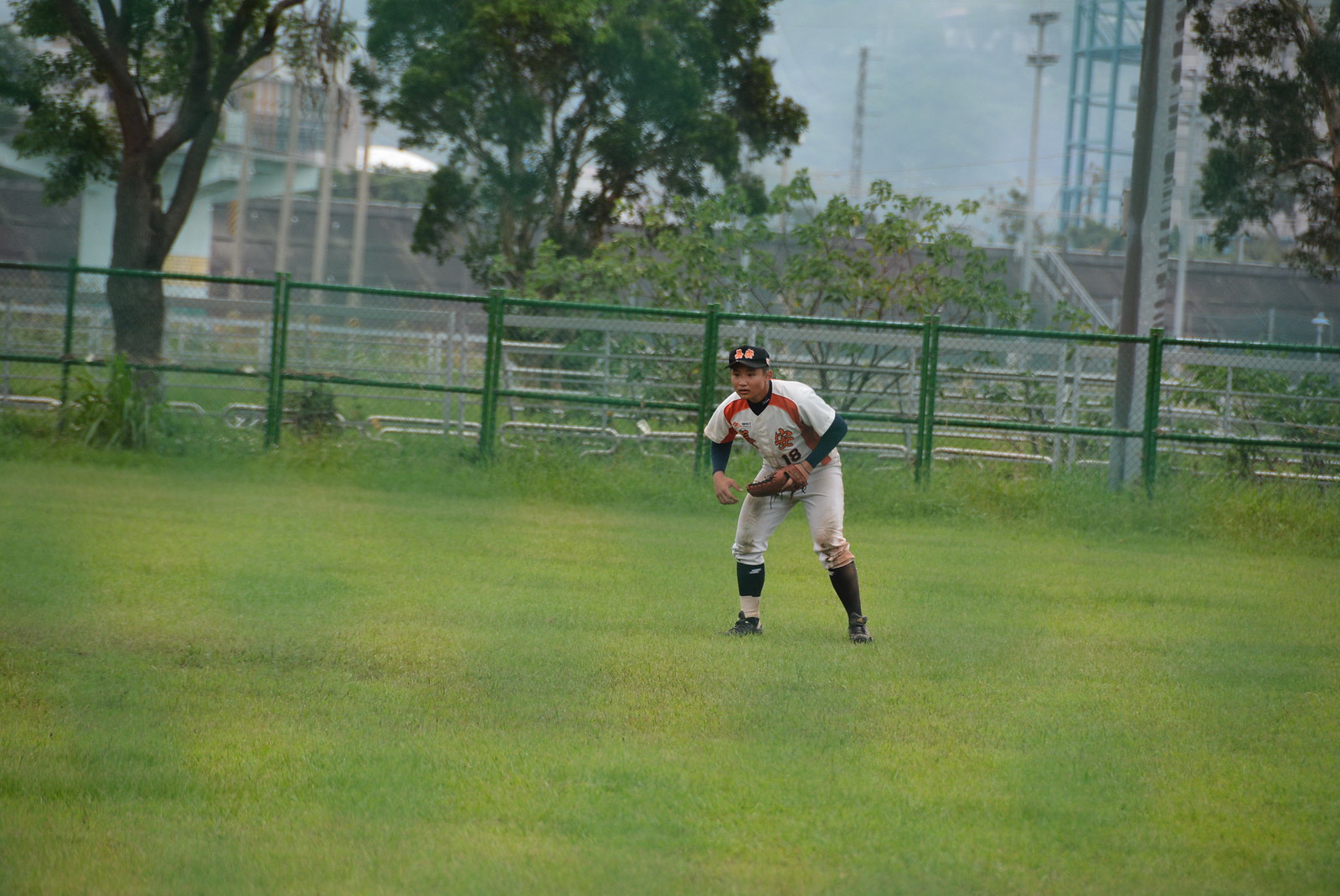The image features a baseball player in a grassy field, surrounded by a mix of natural and man-made elements. The player's uniform is predominantly white with red accents and an orange character on the front, suggesting he might be part of a Japanese team. He wears a black baseball cap adorned with two characters and a green long-sleeve shirt under the jersey. His left hand holds a catcher's mitt, and his attire includes tall black socks and black cleats. There are noticeable dirt stains on his white uniform pants, particularly on the knees and upper thighs. The player is captured in a slightly crouched position, leaning forward with both arms extended, looking intently towards the left angle of the image. 

The setting includes a green, well-maintained grassy area enclosed by a chain-link fence with green posts. Beyond the fence, three trees with dark green leaves and one with lighter green leaves are visible, along with vague structures, a road, and a secondary metal fence farther back. A possible sports stadium with bleachers and a scoreboard is discernible in the background, along with mountainous terrain, light electric poles, antennas, and various towers adding depth to the scene.